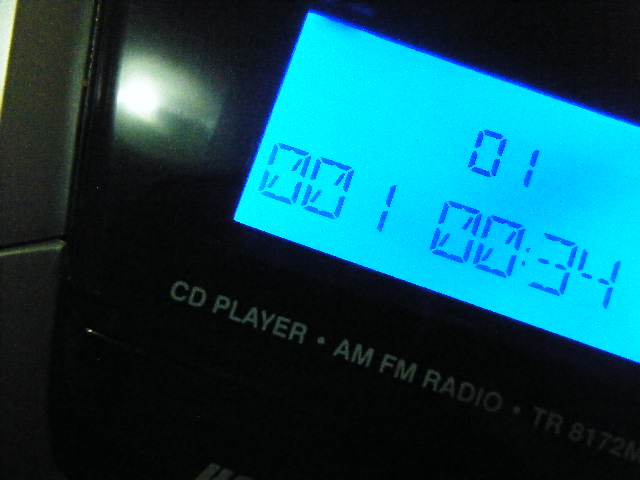This color photograph showcases an in-dash CD player and AM/FM radio unit. The radio appears to be securely mounted within a car's dashboard, with gray, leather-like material partially visible on the left side of the image. The radio and CD player unit features a sleek, shiny black plastic facade, which catches reflections of light. Central to the device is a blue display screen showing the numbers "01" at the top, followed by "001,” and “00-34” beneath it. The model number "TR-8172M" is also visible on the display. Additionally, there is a small blue button located above the main display, adding more functionality to this sophisticated audio equipment.